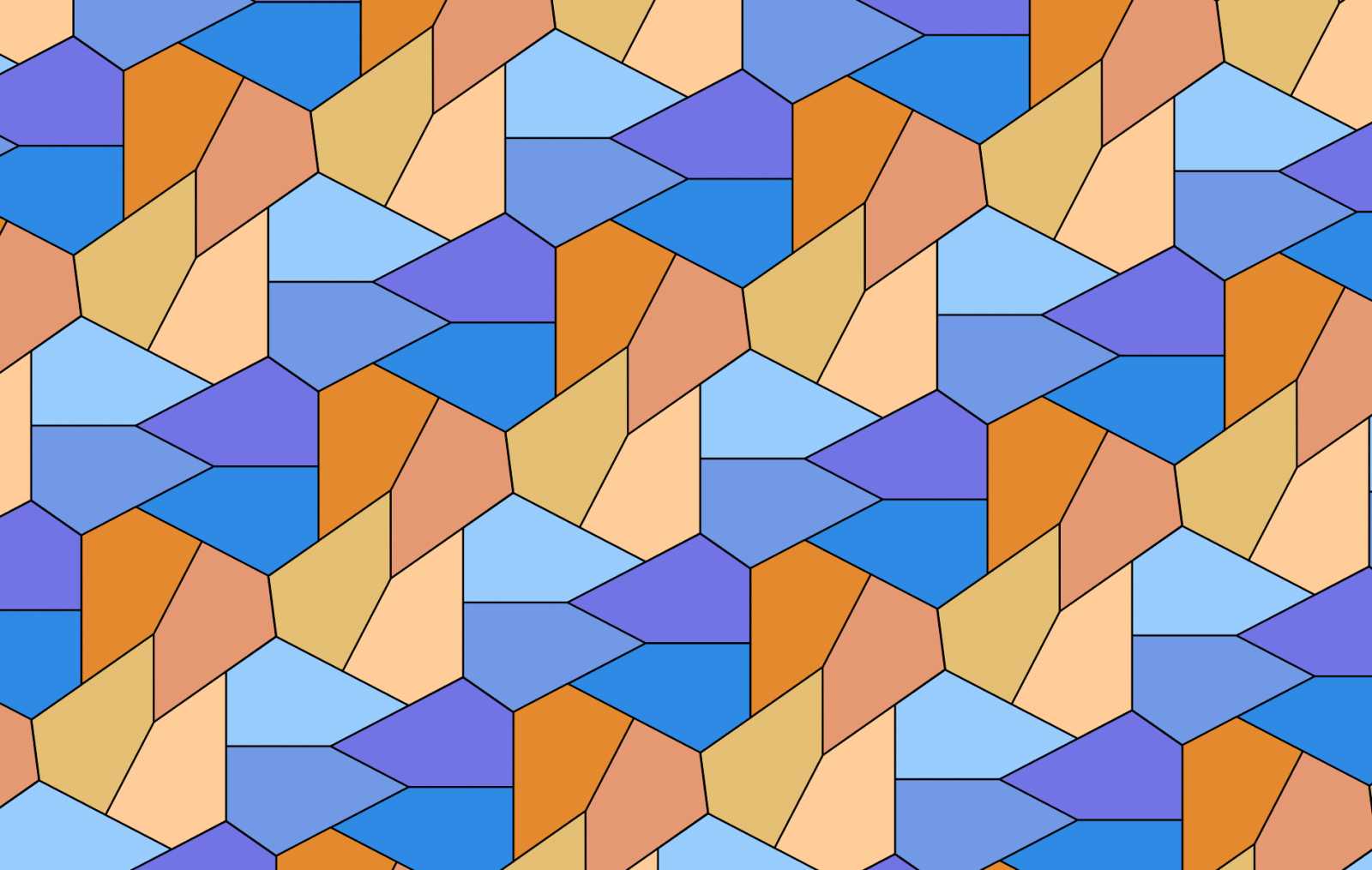The image appears to be a coloring page designed to introduce patterns to children. The intricate design can be colored digitally on a computer or manually using crayons or markers. This busy pattern might also serve as a unique background for a webpage or a scrapbook page.

The page features a repetitive geometric motif that isn't quite triangular. Each shape has a triangular top and side, but the opposite side is flat, creating a unique form when two shapes meet at their flat edges. This forms a four-sided figure with each angle suggesting motion towards the center.

These shapes are organized in pairs and are distinguished by alternating colors. At the bottom, there is a pair consisting of a darker tan and a lighter tan. Facing directly upwards from the flat bottom, two other pairs are made of dark brown and light brown. Adjacent to them are a pair of dark blue and light blue, and another set of colors in a purplish-blue and cornflower blue. The pattern continues in similar groupings across the entire page, creating a visually engaging and repetitive design suitable for educational purposes.